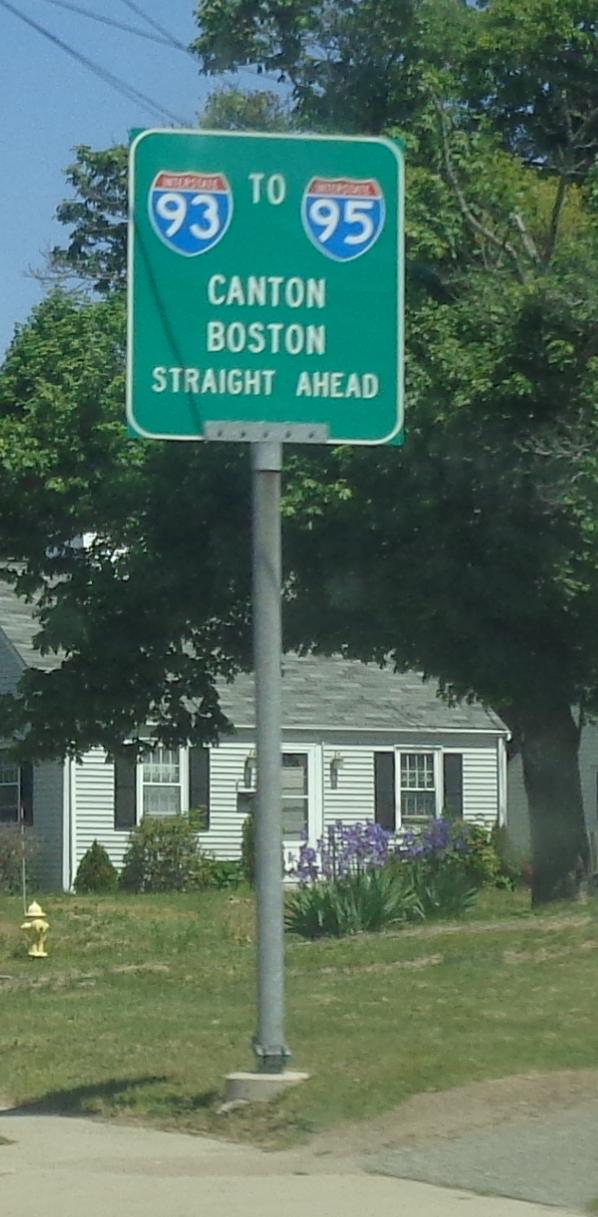This photograph captures a green highway sign indicating directions to Interstate 93 and Interstate 95, as well as to Canton and Boston. The sign is mounted on a stainless steel pole and features distinct red, white, and blue shields for Interstate 93 and Interstate 95. Below these shields, the text "To Canton, Boston" is displayed in white letters, while "Straight Ahead" is noted in a yellowish-green hue. In the background, one can see a white house with white siding and a gray shingle roof, partially obscured by a large tree. At the house's front door, purple lilacs are in bloom, adding a touch of color to the scene.